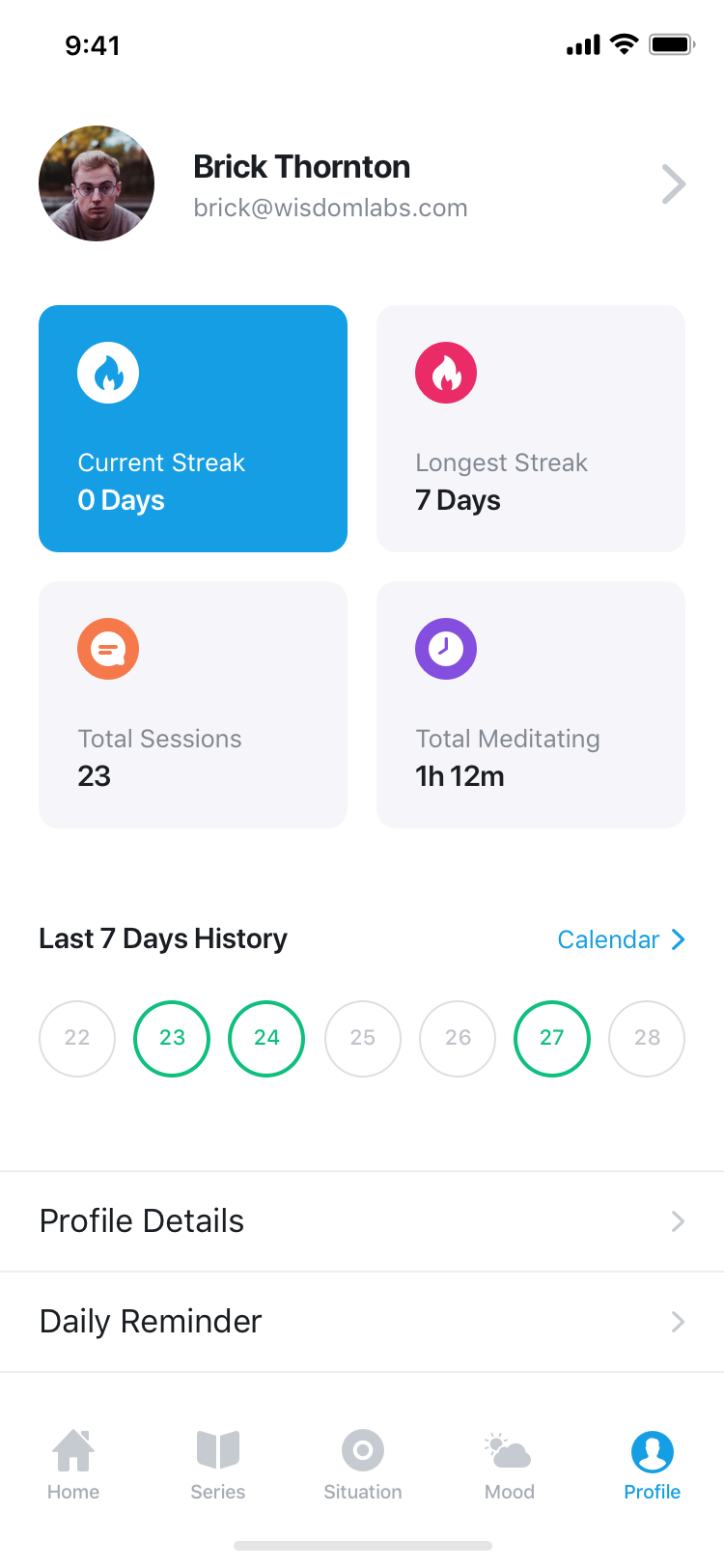Screenshot of a smartphone displaying a wellness app interface. The top of the screen has a white background, with a black status bar showing the time as 9:41, strong signal bars, a Wi-Fi icon, and a fully charged battery. Below the status bar is a user profile section featuring a headshot photograph of the user, Brick Thornton. His name is displayed in bold black letters, and below it, in gray text, is his email address: brick@wisdomlabs.com. There's also a right-facing arrow next to the email address, indicating it is clickable for additional options.

The main interface comprises four rectangular text boxes. The top left box is bright blue with a white circle containing a blue flame icon, indicating "Current Streak: 0 Days." The top right box is white with a red circle housing a white flame icon, showing "Longest Streak: 7 Days." The bottom left box, also white, has an orange circle with a white speech bubble icon and lists "Total Sessions: 23." The bottom right box, white as well, features a purple clock icon and denotes "Total Meditating: 1 Hour 12 Minutes."

Below these statistics, there is a section titled "Last 7 Days History," accompanied by a blue "Calendar" button with a right-facing arrow for accessing a detailed calendar view. The dates displayed range from the 22nd to the 28th, with circles around the dates 23, 24, and 27 in green, indicating the days the user engaged with the app.

Following this section, there are expandable menu options for "Profile Details" and "Daily Reminder," each with a right-facing arrow.

At the bottom of the screen, there are navigation icons for "Home," "Series," "Situation," "Mood," and "Profile," with the "Profile" icon currently selected.